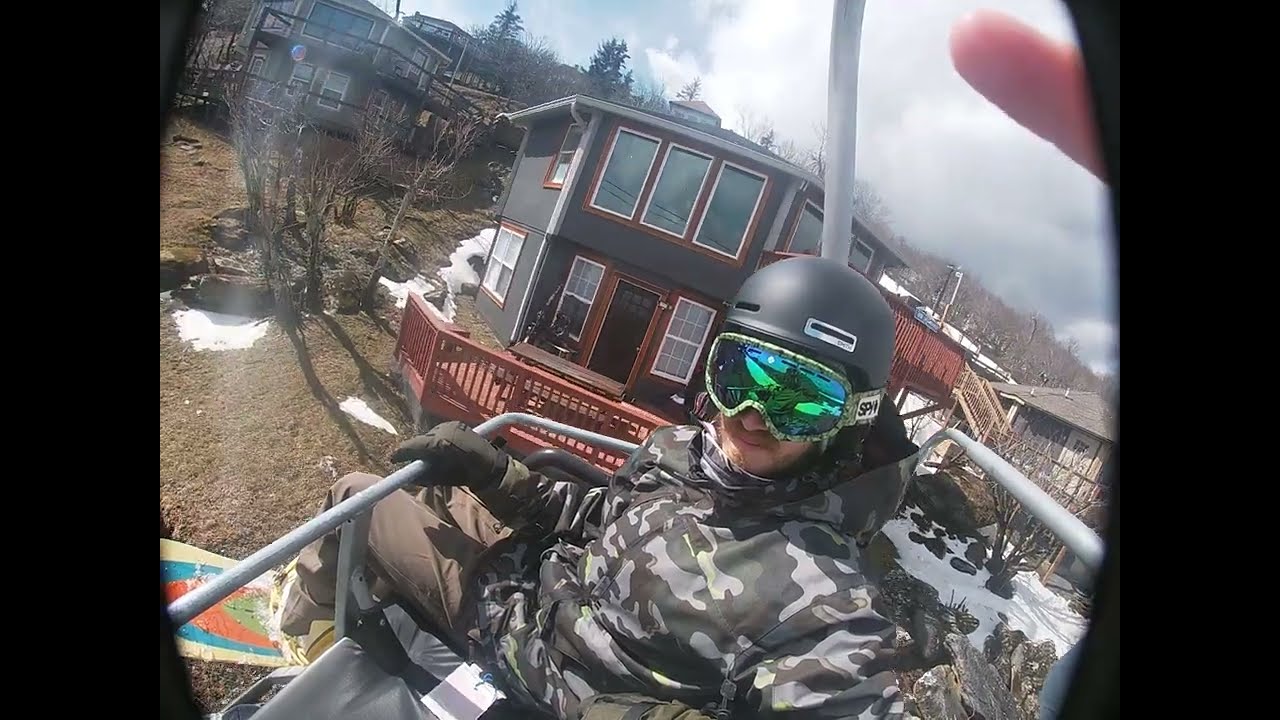The image captures a man seated on a ski lift, his snowboard securely fastened to his feet. He is dressed in a black and gray camouflage ski jacket with a hood, beige pants, and substantial black gloves. His head is protected by a smooth black matte helmet adorned with reflective greenish-blue goggles. The man is holding on to the ski lift's pole and looking directly at the camera. Surrounding him in the backdrop, the scene unfolds into a winter landscape dotted with houses nestled on the side of a hill. The house closest to the ski lift features an octagonal shape, spans two stories, and has a large deck with a picnic table in front as well as another smaller deck behind it. Additional houses are visible scattered across the hillside, with barren trees interspersed, conveying a wintry atmosphere. Unique to this photograph are black side panels, hinting that the image might be taken through a narrow viewpoint or peephole, and a glimpse of a finger intrudes on the upper right corner, adding an element of candidness to the shot. Small patches of snow on the ground and a target-like pattern featuring white, blue, red, and green colors in the lower left contribute to the enigmatic and detailed composition of this winter scene.